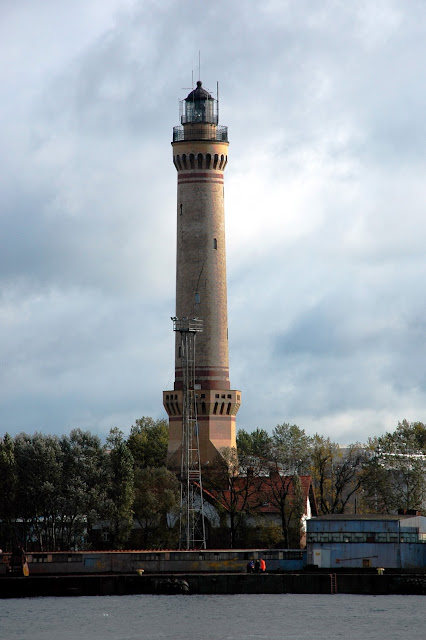This vertical photograph captures an outdoor scene centered around a tan, brick lighthouse with a black top and a series of windows and a gate near the top, resembling a minaret in design. The lighthouse is located at the end of a dock that supports a smaller, dilapidated building, painted in blues and grays, possibly with broken windows and topped with a radio antenna. In the foreground, there is water, suggesting the photo was taken from this vantage point. Before the lighthouse, you notice a small white house with a red roof, partially hidden by green trees indicating a spring day. To the left and right of the lighthouse, you see additional buildings and lush treetops, all set against a cloudy, blue sky. The scene seems to include a railway, or perhaps an old train station, situated near rusted buildings with corrugated roofs. Overall, the image exudes an atmosphere of serene neglect, with nature and weathered human structures coexisting harmoniously.